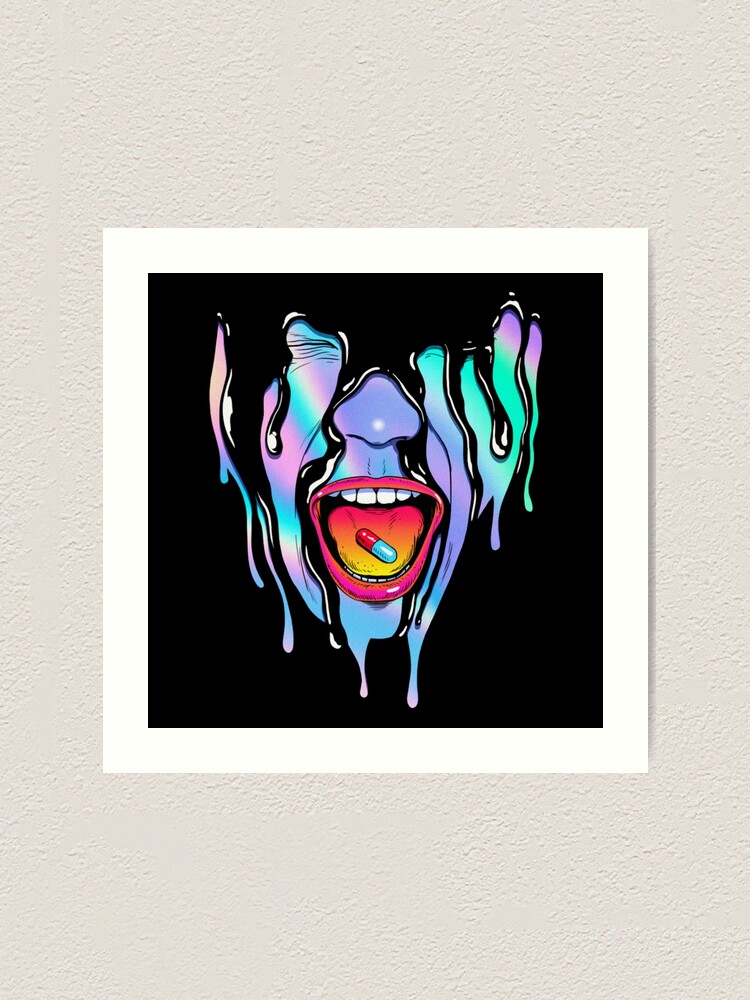The image is a modern art painting set against a black background, matted with a white border, and displayed on an off-white stucco wall. The painting focuses on the bottom half or two-thirds of a person's face rendered in striking shades of purple and blue, mixed with hints of teal and pink. The mouth is open wide, revealing white teeth and a vivid red and yellow tongue. Centered on the tongue is a red and blue capsule. The face appears to be in a state of distress or duress, as suggested by the rivulets and droplets of black ink, along with additional blue and purple pigments, dripping down from the face. The person's eyes are squeezed shut, reinforcing the sense of distress.